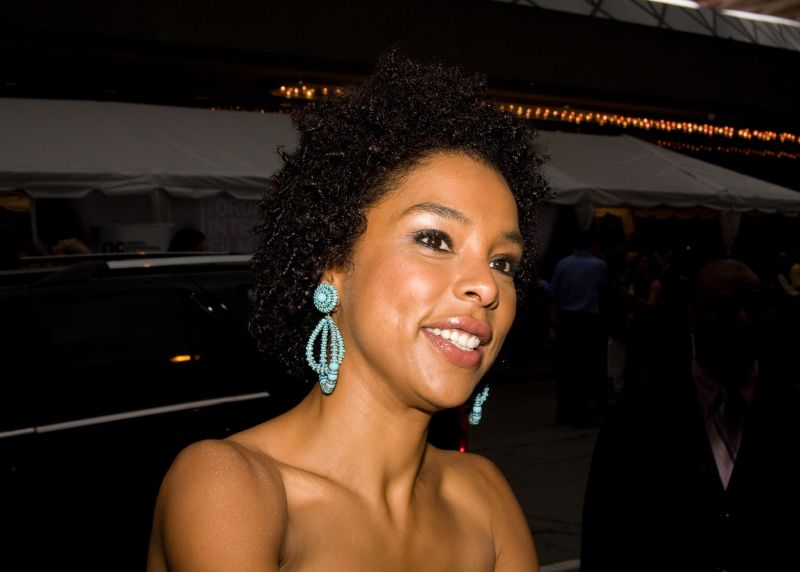In this image, a young black woman is the focal point, captured from her shoulders up. She has short to medium-length curly hair and is donning beaded turquoise earrings, featuring a large circular part connected to dangling beads. Her shoulders are bare, suggesting she might be wearing a strapless top. The woman is smiling gently and gazing slightly to the right. The background is predominantly dark, likely taken with a flash, and features a white tent and string lights, hinting at an event setting with other people scarcely visible. The overall scene suggests a lively atmosphere, but the emphasis and light are solely on her, highlighting her joyous expression and detailed accessories.